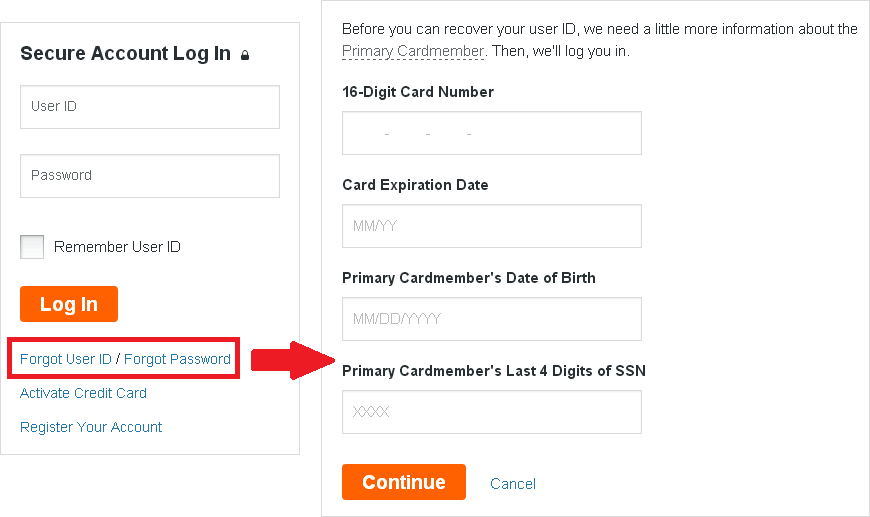**Caption:**

The image features a side-by-side comparison of two screens from a secure login portal. 

- **Left Side:**
  - The left screen depicts a standard login interface.
  - At the top, a small padlock icon signifies a secure page.
  - Below, there are input fields for "User ID" and "Password."
  - A checkbox marked "Remember User ID" is situated beneath the password field.
  - Prominently displayed is an orange "Login" button.
  - Additional options include:
    - "Forgot User ID"
    - "Forgot Password"
    - "Activate Credit Card"
    - "Register Your Account"
  - The options "Forgot User ID" and "Forgot Password" are emphasized within a red-highlighted box, and an arrow directs attention to the adjacent screen.

- **Right Side:**
  - The right screen provides a step for recovering User ID or password.
  - The header reads: "Before you can recover your User ID, we need a bit more information about the primary cardholder."
  - Fields include:
    - "16-Digit Card Number"
    - "Expiration Date"
    - "Primary Cardholder’s Date of Birth"
    - "Primary Cardholder’s Last Four Digits of Social Security Number"
  - At the bottom, options to "Continue" or "Cancel" complete the interaction.

This detailed comparison illustrates the process and required information to recover a forgotten User ID or password for the secure login portal.